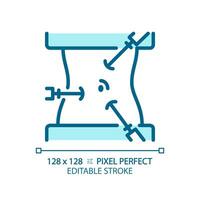This image appears to be a diagram likely intended for a textbook, illustrating the spatial relationships between pixels. The central figure is shaped somewhat like an egg timer, featuring light blue coloration at its top and bottom. From various points around this figure, arrows or needle-like indicators point towards the center from the left, top right corner, and lower right corner, each resembling a needle with a curved arc at the end. The middle of the diagram contains a dot and an arc arranged in a way that resembles an eye and an eyebrow. There is also a thin line spanning across the image, with a square at each end. At the bottom of the image, small text reads, "128 by 128 equals pixel perfect, editable stroke."